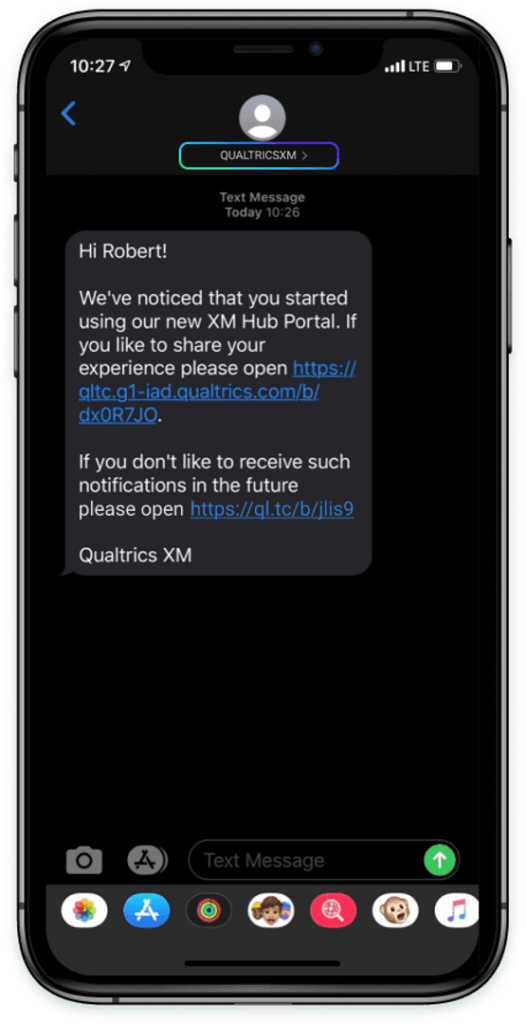In this photo captured from a cell phone screen, we see a text message, partially visible under a small profile icon that resembles a face. The sender's name is obscured, but the message clearly displays the date and time: "Today at 10:26 AM". The content of the message is as follows: 

"Hi Robert, we've noticed that you started using our new XM Hub portal. If you'd like to share your experience, please open [link]. If you don't like to receive such notifications in the future, please open [link]. Qualtrics XM."

Below the message, the interface allows the recipient to respond, indicated by a text input field and "Text Message" instructions. Additionally, a row of app icons is visible, featuring symbols that include a search icon, a flower, a triangle, and a face. The exact nature of these icons is unclear, suggesting it might be an iPhone interface, which may be unfamiliar to the reviewer.